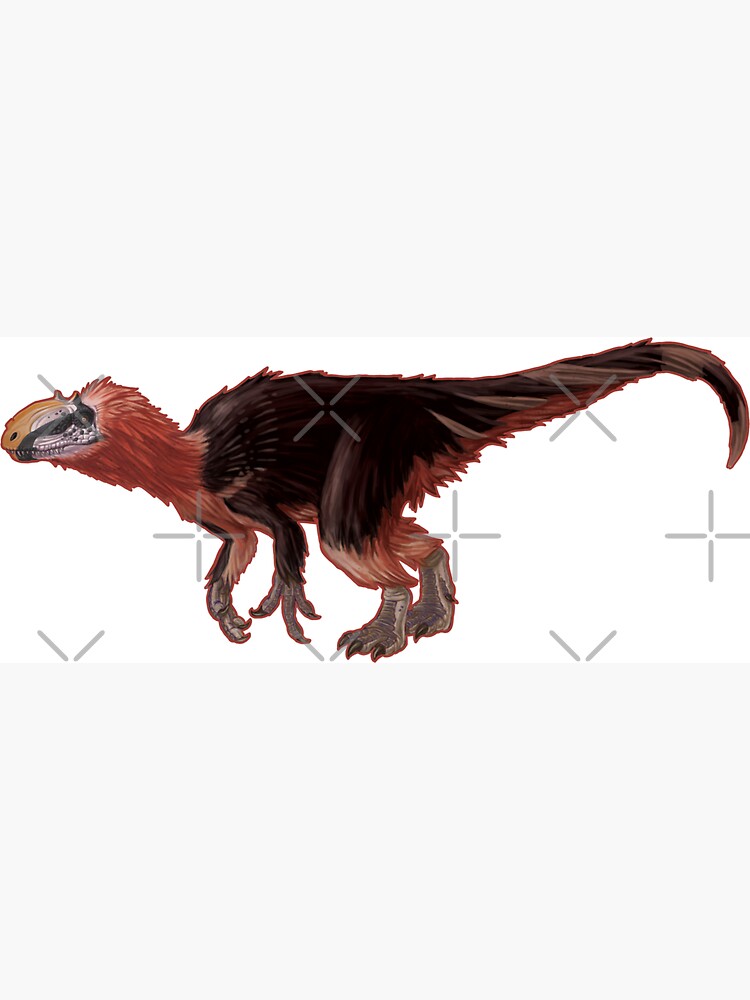This image appears to be a highly detailed and stylized drawing from a children's book, depicting a creature that is a combination of a dragon and a dinosaur. The creature features a blend of dinosaur and bird-like characteristics, with a long, graceful tail that curves downward and ends in a point. The body is covered in a mix of fur and feathers, predominately black and light brown, with rough feathers accentuating its back and neck.

The creature’s head is a focal point, with a yellowish face adorned with a distinctive black stripe running across its eye. It possesses a long, curved nose ending in visible white teeth, giving it a slightly fierce appearance. The neck is colored in a reddish-brown hue, seamlessly blending into the body. Tiny nubs resembling horns protrude from the top of its head, adding to its mythical aura.

Its muscular forearms, which end in three gray fingers tipped with black claws, are highlighted by red on their inner parts. The forelimbs hang in front, reminiscent of a Velociraptor's poised stance. It’s equipped with two powerful hind legs, also ending in three black-clawed toes, showcasing greyish tones towards the feet. The legs appear sturdy, supporting the creature’s dynamic posture.

The upper body is predominantly covered in brown feathers, while the underside displays a reddish peach tint extending to the arms and neck. The juxtaposition of these colors adds to the creature's vibrant and animated look. Overall, this meticulously crafted creature melds elements of prehistoric and fantastical, captured in a striking side view that brings its vivid details to life.